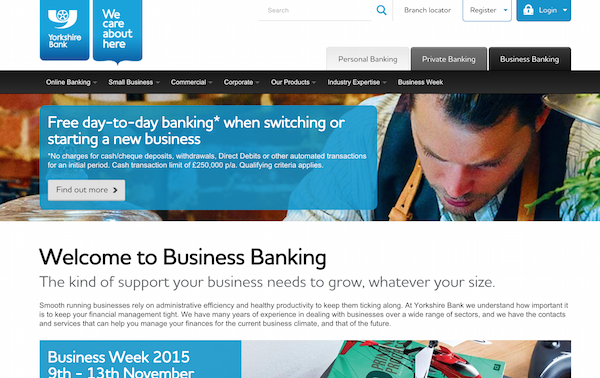This image showcases the homepage of the Yorkshire Bank website, which features a white background adorned with a harmonious blue, black, and white color scheme. At the top left, two prominent blue boxes capture attention. The first box displays the "Yorkshire Bank" text alongside the bank’s logo, while the adjacent box bears the slogan "We care about here."

Towards the top right corner, a set of functional elements are neatly arranged, including a search bar, a branch locator link, and options to "Register" and "Login." Below, three banking categories are presented in distinct shades: light grey for "Personal Banking," darker grey for "Private Banking," and black for "Business Banking."

A long horizontal navigation bar extends across the page, offering various menu options. From left to right, it includes links to "Online Banking," "Small Business," "Commercial," "Corporate," "Our Products," "Industry Expertise," and "Business Week," with dropdown menus available for all except the latter.

Beneath the navigation bar, a large banner image featuring a person at work provides a dynamic backdrop. Superimposed on this banner is a sizable, light blue rectangular box containing white text that advertises, "Free day-to-day banking when switching or starting a new business." A prominently placed white button below the text invites users to "Find out more."

Following this, a section of white space is occupied by welcoming text that reads, "Welcome to Business Banking – the kind of support your business needs to grow, whatever your size," accompanied by a brief summary. 

Lastly, another background image with a partially visible blue box announces "Business Week 2015," slated for November 9th to 13th, though some text is cut off.